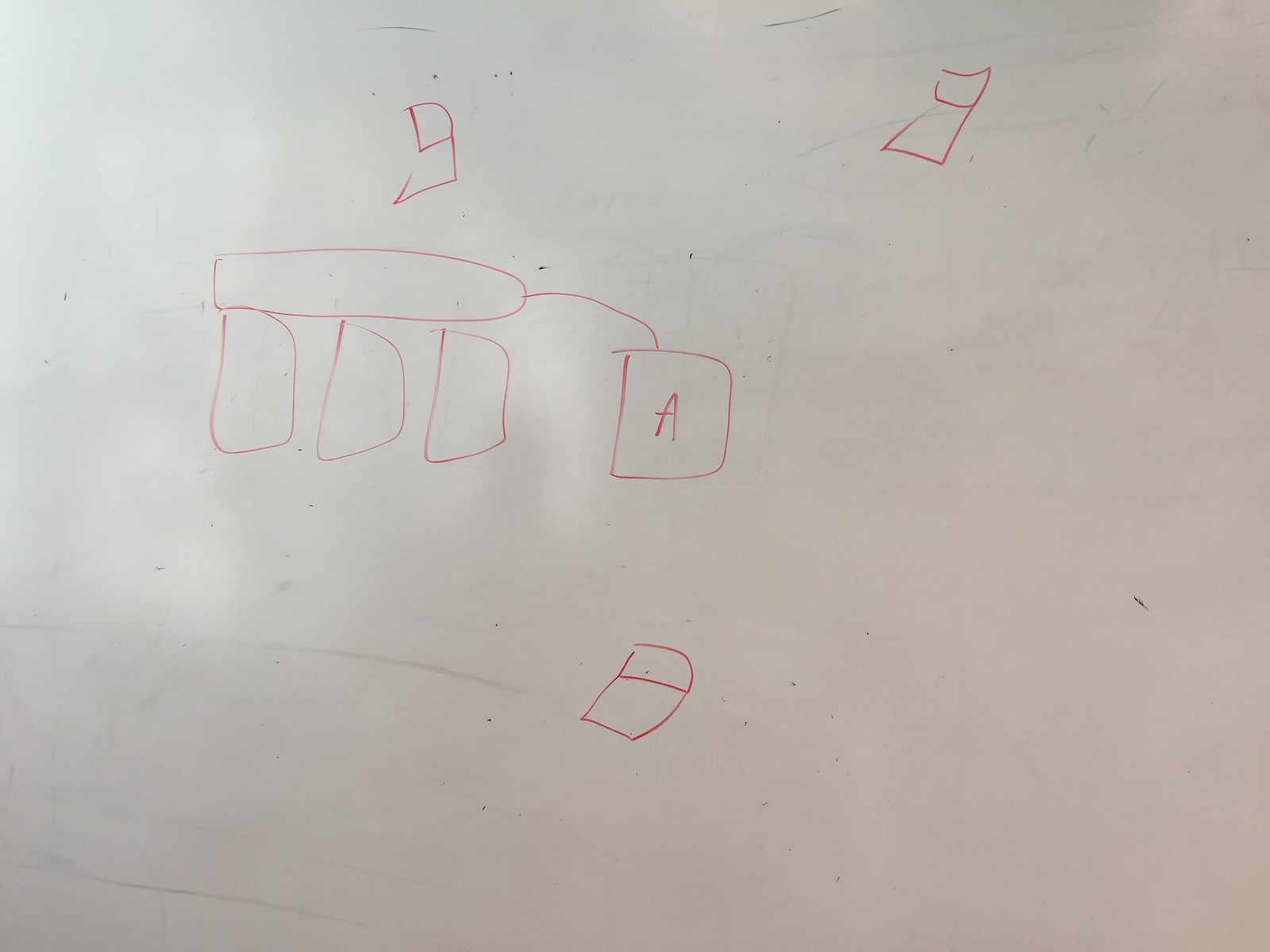This is a detailed pencil sketch on a piece of white paper that has a subtle pink tint. The artist has used a red ink pen to doodle a variety of objects. Dominating the center of the page is a long cylindrical block, supported by three smaller brown blocks, reminiscent of a stonehenge-like structure. Extending from one end of the cylinder is a curvy line leading to a square box, which contains the letter "A" inside it. Below this square box, there's a doodle that resembles the shape of a lonely bee. Additionally, there are other elements on the upper part of the paper. One bee-shaped drawing is positioned directly above the stonehenge structure, while another letter-like "B" doodle is in the top right corner. These upper doodles are isolated and don’t connect with any other elements on the paper.